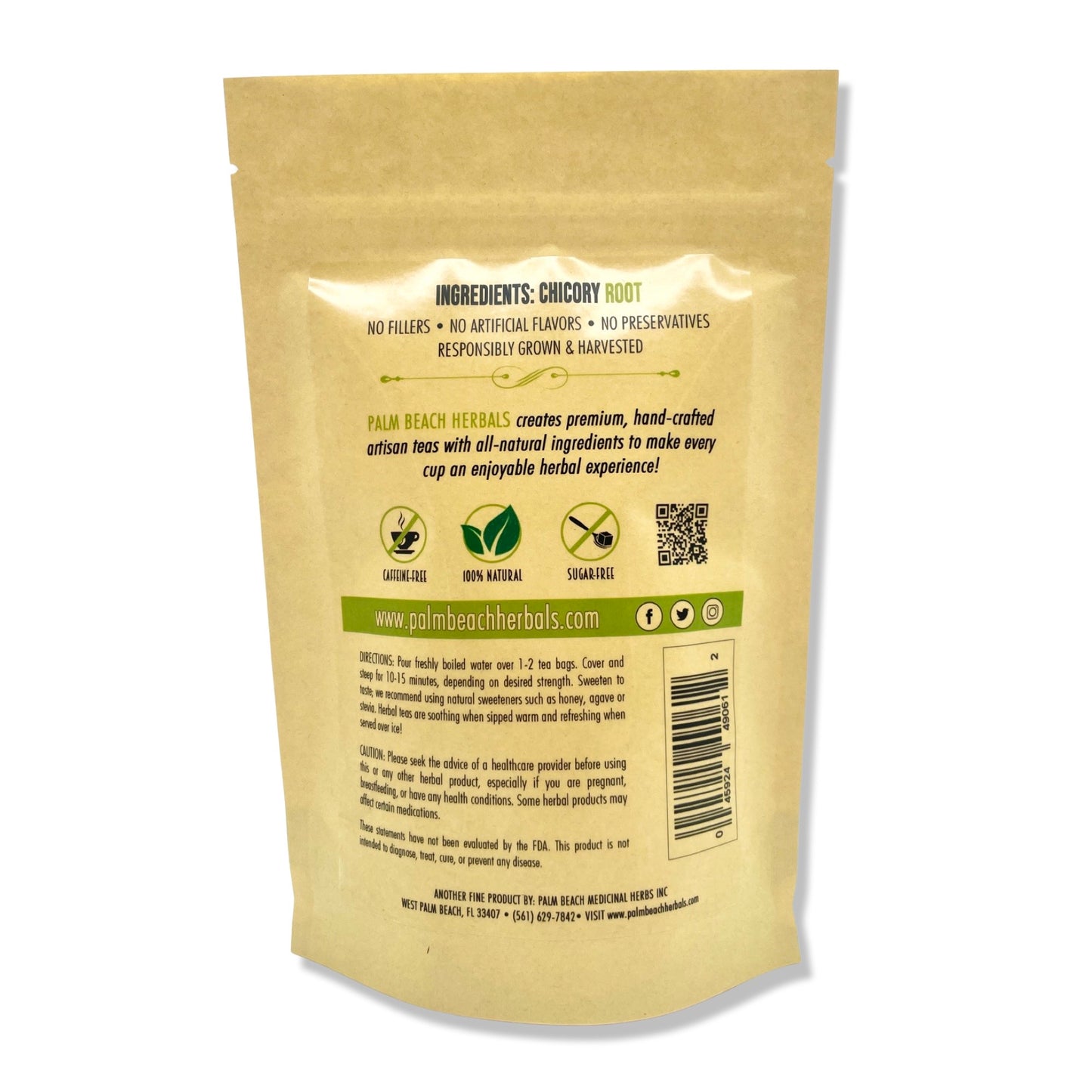This image showcases the back of an unopened, brown paper supplement bag, likely from a brand similar to Anthony's Fiber, commonly available on Amazon. The bag prominently features the product's solitary ingredient: chicory root. The packaging, from Palm Beach Herbals, emphasizes its commitment to purity with claims of no fillers, no artificial flavors, and no preservatives, all responsibly grown and harvested. It also highlights the product's benefits with clear symbols indicating it is caffeine-free, 100% natural, and sugar-free. A QR code is visible alongside the company's website, www.palmbeacherbals.com. Additionally, the bag offers detailed information about the company's dedication to creating premium, handcrafted artisan teas, aiming to provide an enjoyable herbal experience. Below these details are instructions for preparation, cautions, and smaller texts, ending with a barcode on the right side.